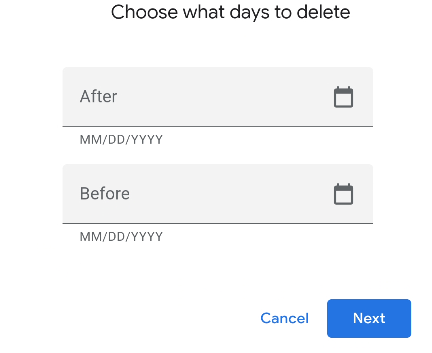The image displays a mobile website with a minimalist design. The page presents a user with options to select specific dates for deleting content. It features prominently two fields for the user to choose the period they want to delete: either through a clickable calendar interface or by manually entering dates in the MM/DD/YYYY format. Users can specify exact dates for deletion by selecting "Before" or "After" a particular date. There are action buttons at the bottom allowing the user to either cancel the operation or proceed by clicking "Next". This functionality seems useful for scenarios such as selectively deleting photos – for example, a user wishing to delete all content after July 1st or before May 31st, thereby retaining only photos taken during a June trip.